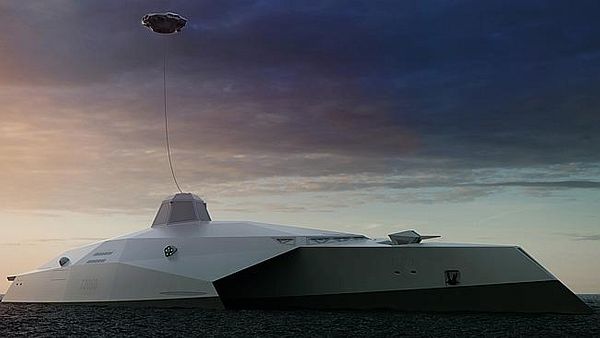This detailed photographic image depicts a futuristic military vessel in an outdoor setting with a unique and unconventional design. The ship features a downward-sloping front reminiscent of a submarine and is entirely enclosed without visible windows, save for a thin opening at the roof. This tapered roof is triangular to rectangular in shape. Dominating the rear of the vessel is a dome or tower from which a thin cable extends, holding a balloon-like apparatus aloft, likely an antenna. On the roof at the very front of the ship, there's a small protrusion resembling a cannon or antenna. The background moodily transitions from dark, cloud-laden skies to patches of light blue, suggesting an early morning or dusk atmosphere.